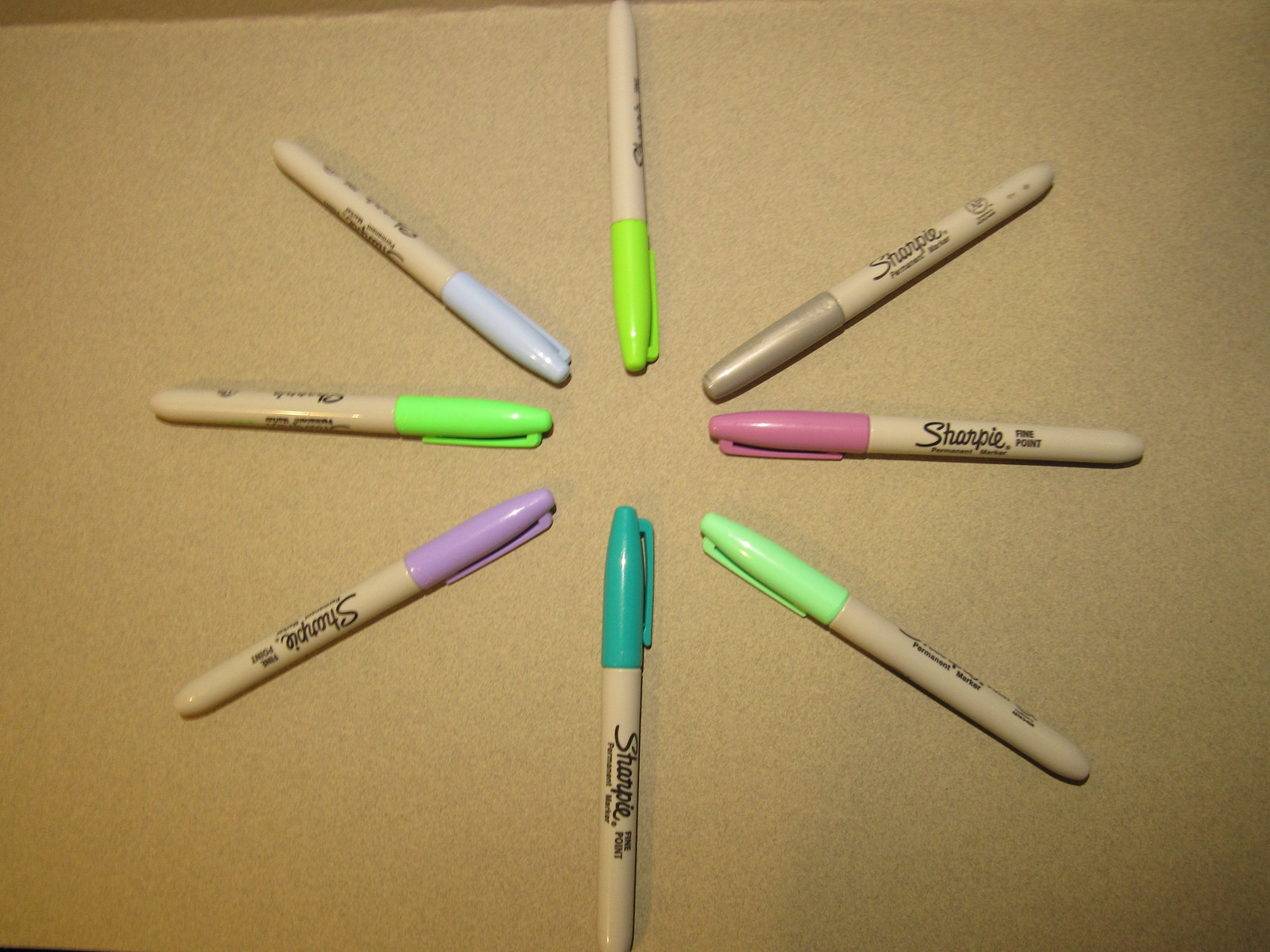This photograph captures a neatly arranged collection of eight Sharpie markers set against what appears to be a brown, possibly cardboard surface. The lighting, likely from a ceiling light, casts hard shadows and provides a slight reflection off the caps, indicating an indoor setting, possibly someone's home. The markers, identifiable by the "Sharpie fine point" branding on their bodies, are uniformly arranged in a circular, star-like pattern with their caps pointing inward.

The colors represented include pastel shades of green, pink, blue, purple, and a distinct seafoam green, along with a pastel purple and periwinkle. Additionally, there are two shades of teal, a vibrant neon green, silver, and a dark purple, making the arrangement visually appealing with its soft palette. The careful arrangement of the markers, coupled with the detailed color variety and lighting effects, creates an aesthetically pleasing and well-organized display of these pastel Sharpies.